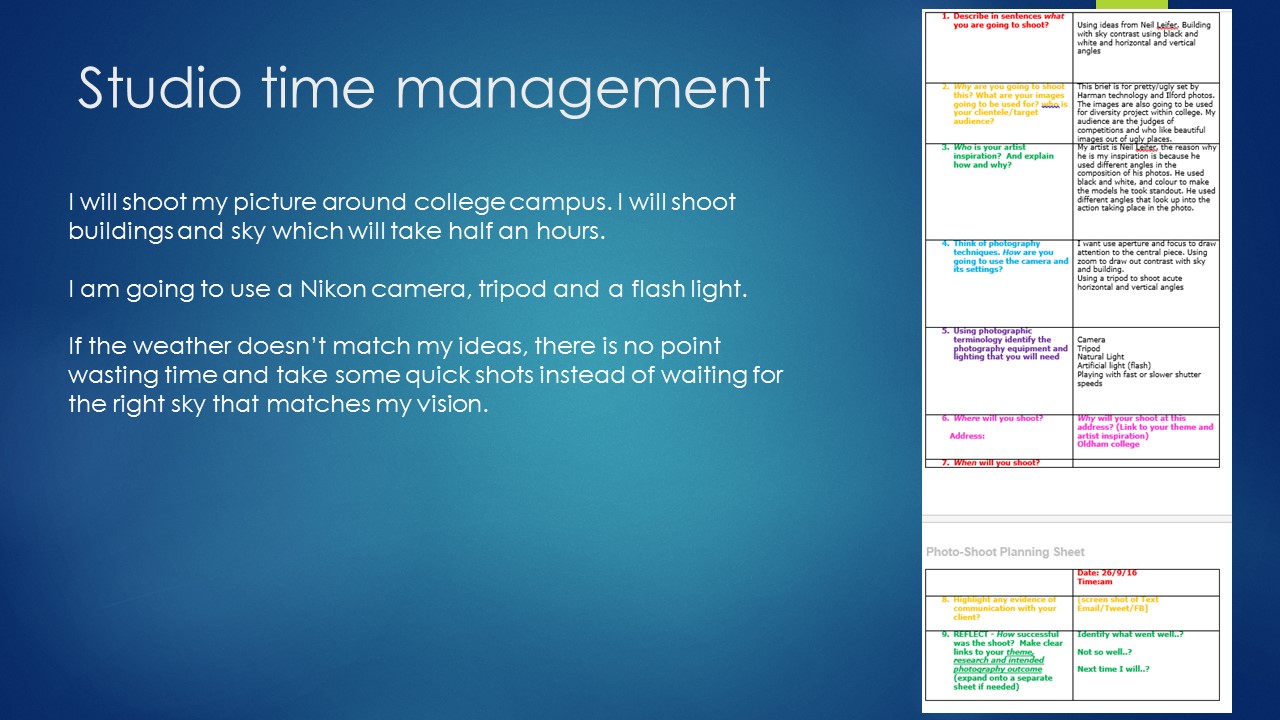The image is a slide from a presentation with a radial gradient background, transitioning from a dark blue at the edges to a lighter blue at the center. The title "Studio Time Management" is prominently displayed in white text at the top left. Below the title, the text reads: "I will shoot my picture around college campus. I will shoot buildings and sky, which will take half an hour. I'm going to use a Nikon camera, tripod, and a flashlight. If the weather doesn't match my ideas, there is no point in wasting time; I'll take some quick shots instead of waiting for the right sky that matches my vision." On the right side of the slide, there is a detailed spreadsheet or chart. It comprises two columns with five rows each, forming a grid of ten boxes in total, with a smaller chart below it consisting of two columns and two rows. The chart contains various colored texts and appears to outline a schedule or plan for the shoot.